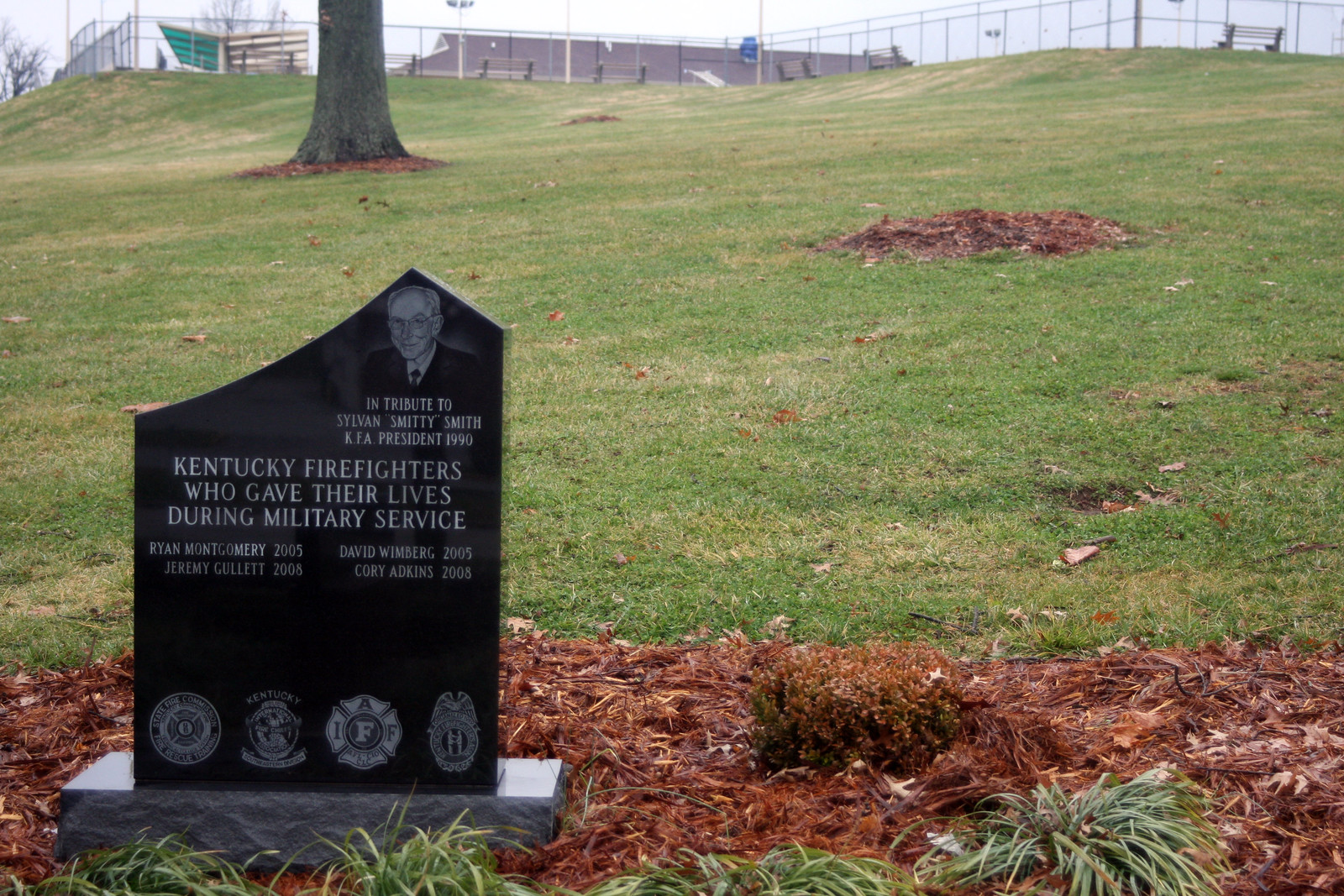The image depicts a meticulously maintained memorial situated in what appears to be an open green field or a garden-like setting. The central feature is a black headstone with an etched, lopsided roof design, serving as a monument. The face of the headstone features a smiling older man with glasses, bald with gray hair, dressed in a black suit with a shirt and tie. This image accompanies the inscription: "In tribute to Sylvan 'Smitty' Smith, KFA President 1990." Below this, the text pays homage to "Kentucky firefighters who gave their lives during military service" and lists the names: Ryan Montgomery (2005), Jeremy Gullett (2008), David Wimberg (2005), and Corey Adkins (2008). The monument is surrounded by well-groomed brown mulch and a pruned shrub, indicating recent landscaping. In the background, there is a tree, a lush expanse of grass, and a distant building with a chain link fence enclosure, suggesting a serene, possibly park-like or cemetery setting.